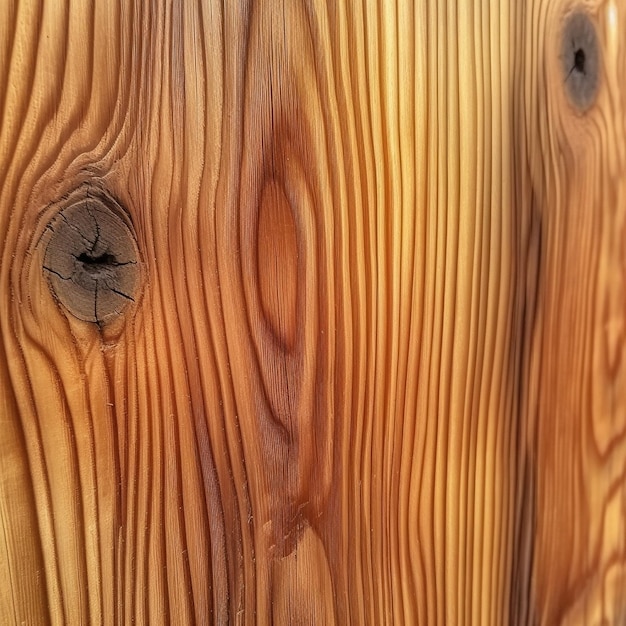The image portrays a close-up of a piece of polished and stained wood in portrait mode, filling the entire frame. The wood exhibits a rich array of colors, ranging from light brown to caramel, with hints of yellow, pink, and even orangish-umber streaks. The most prominent feature is a large, natural knot located slightly above the center on the left-hand side. This knot is characterized by a dark brown spot at its core, surrounded by wavy lines and cracks, transitioning back into the regular wood. Another knot is visible at the top right-hand corner, although it is blurred; this knot has a black center encircled by gray lines. The gradations and natural lines of the wood are vivid and detailed, highlighting the texture and imperfections, such as ridges and crevices. This wood could be used for various purposes, such as paneling or furniture making.